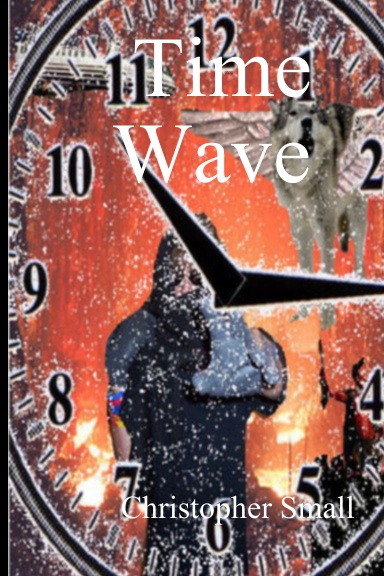The image is a detailed and somewhat worn book cover with a rustic, reddish-brown color scheme reminiscent of aged wood. The title "Time Wave" is prominently displayed in large white letters at the top, while the author's name, "Christopher Small," appears in smaller white text at the bottom. Dominating the image is a close-up view of a partially visible clock face, with the hour hand pointing near the 11 o'clock mark and the minute hand at 3 o'clock. Superimposed in the middle of the clock is the enigmatic figure of a man dressed in black, wearing sunglasses, and extending his hand towards the viewer. Adding to the surreal elements, the upper right part of the clock face features a winged wolf. The intricate details, like the blimp and the mix of rustic and fantastical elements, suggest a mysterious and possibly time-related narrative.